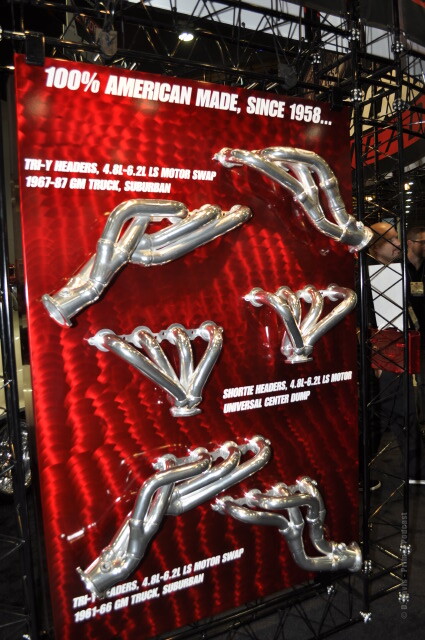The photograph depicts a convention display featuring a vibrant red billboard secured to a metal grid frame. Prominently, at the top of the sign in bold white font, it states, "100% American Made Since 1958." The display showcases six 3D chromed engine parts intended for various automotive applications. These parts are organized into three distinct types, with two examples of each type. The specific parts are labeled as Tri-Y headers for 4.6 liter to 6.2 liter LS motor swaps (fitting 1967-87 GM Trucks and Suburbans), Shorty headers, and Motor Universal Center Dump headers, with descriptions in white text next to each one. The scene is set against a black grid and appears busy with convention attendees in the background, including several men in black shirts, enhancing the bustling atmosphere.